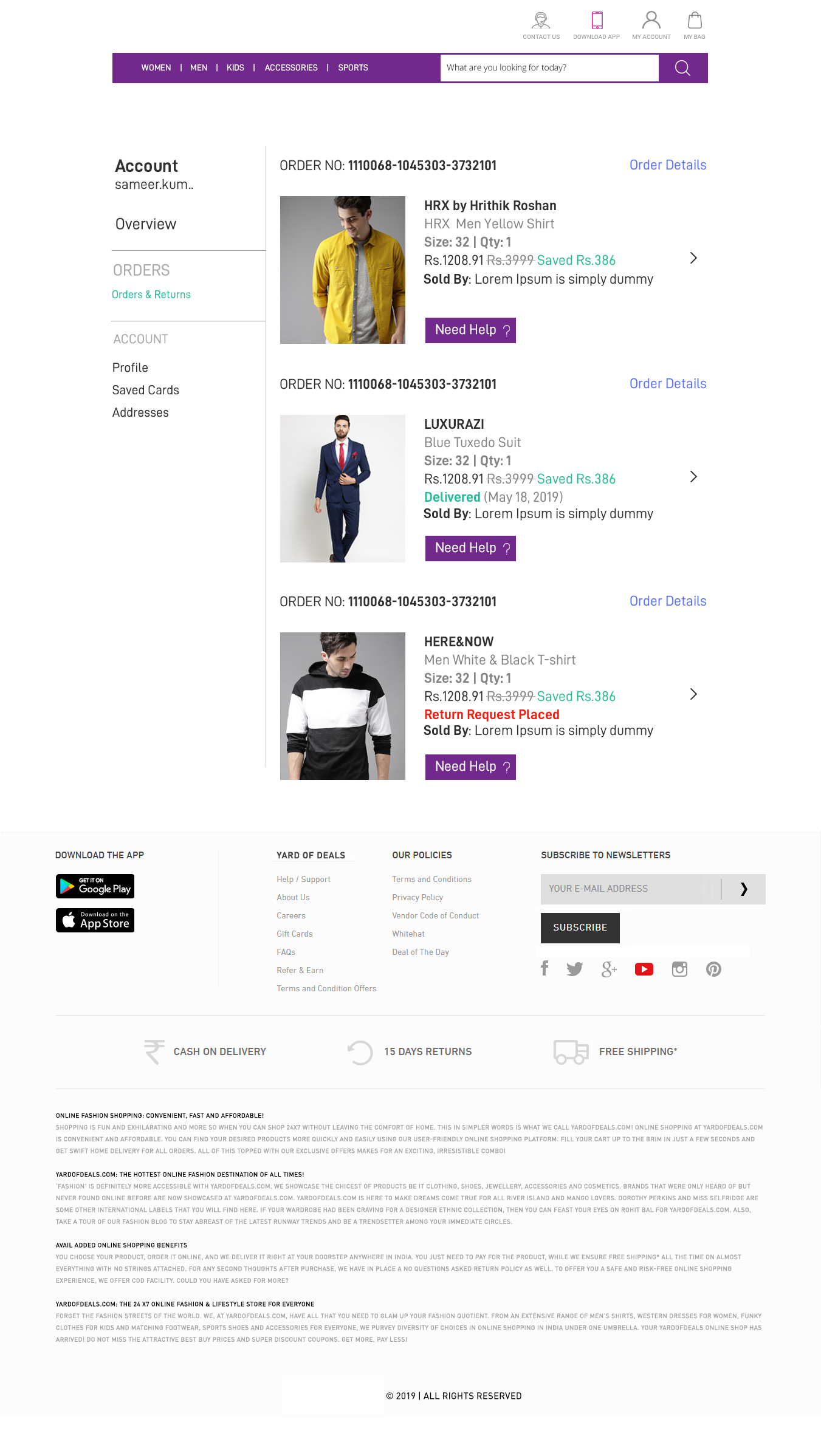The screenshot showcases an online shopping website with a prominent purple navigation bar at the top that includes categories such as "White Texas Women," "Men," "Kids," "Accessories," "Sports," and various utility options like "Contact Us," "Download App," "My Account," and "Bag." A magnifying glass icon is present for search functionality. 

On the left side is a sidebar starting with the bold heading "Calm, Start" in black letters. The sidebar contains various account management options, including "Sameer.com," "Orders," "Orders and Returns," "Account," "Profile," "Save Cards," and "Addresses."

The main section details a specific order with the Order Number: NL-1110068-1045303-3732101. The order includes an item labeled as "HRX Men Yellow Shirt," size 32, priced originally at RS-1208.91 but discounted to RS-399, with the savings highlighted in blue as "Saved RS-386." The vendor is listed as "Simply Dummy." 

Another item in the order is a "Lex Rossi, Blue Tuxedo Suit," also size 32, priced at RS-386. Below these details are promotional text and links encouraging users to download the app from Google Play, explore deals, seek help, and look into terms of service and privacy policy. The page concludes by highlighting the benefits of online fashion shopping, described as convenient, fast, and affordable, marking the site as a top fashion destination. 

Overall, the site emphasizes user convenience and a streamlined shopping experience with a focus on fashion items and significant savings.